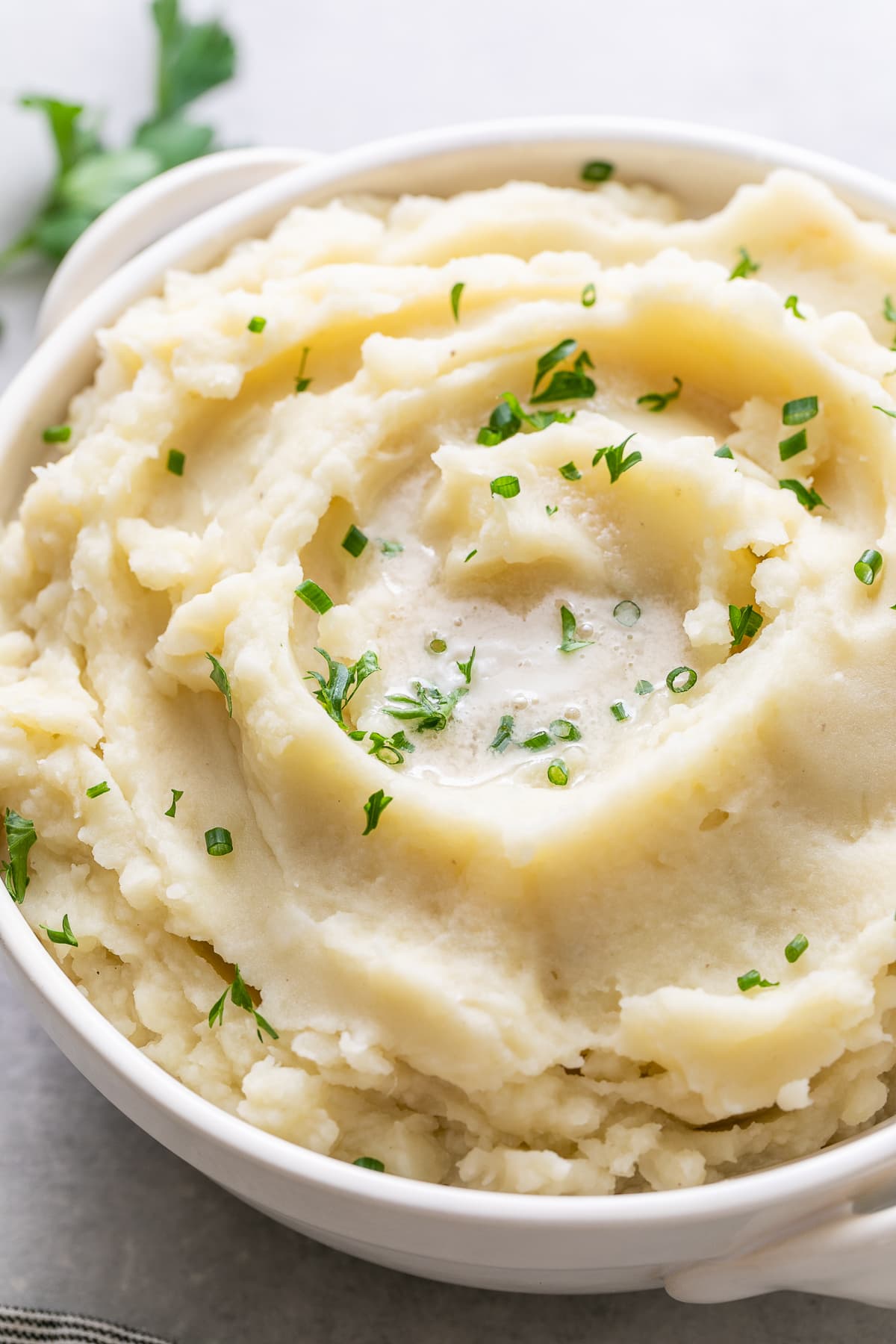In a bright, pristine photograph with a slightly blurry, indeterminate background, a white bowl takes center stage. The bowl, round with a subtle handle on one side, sits prominently on a white table. The top view reveals a generous serving of creamy, fluffy mashed potatoes, artistically swirled into a circular pattern that peaks at the center, showcasing its smooth and airy texture tinged with a yellowish, off-white hue. Sprinkled atop the potatoes are finely cut green chives, adding a fresh contrast to the creamy expanse. Just beyond the bowl, at the top edge of the image, a green leaf peeks into the frame, and a barely visible fabric napkin rests to the left, enhancing the simple, inviting composition.